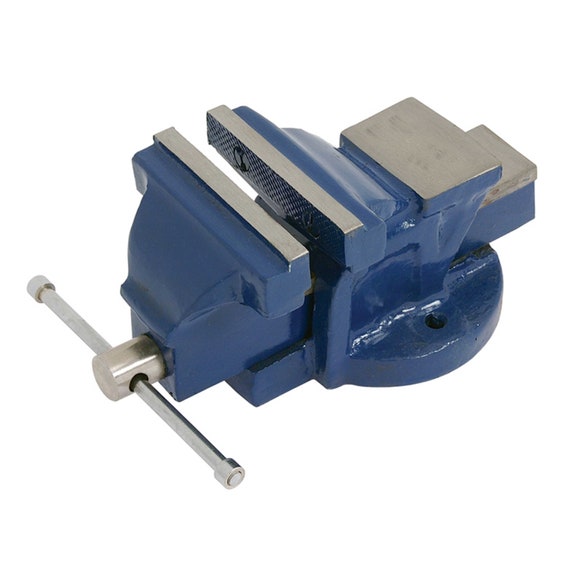The image depicts a dark blue metal vise, commonly used on a workbench to securely hold objects in place. The vise features a body painted in dark blue with brushed silver components, including the crank handle, jaws, and other metal parts. The vise has two front handles for tightening or loosening its grip. Notably, two holes are visible on the base, allowing it to be bolted to a workbench for added stability. At the back of the vise, there's a flat anvil surface suitable for hammering tasks. The left side houses a long, split handle, while the top consists of two flat, silver metal jaws with inner divots, designed for gripping items securely. The overall structure is a blend of silvery metal and dark blue painted surfaces.